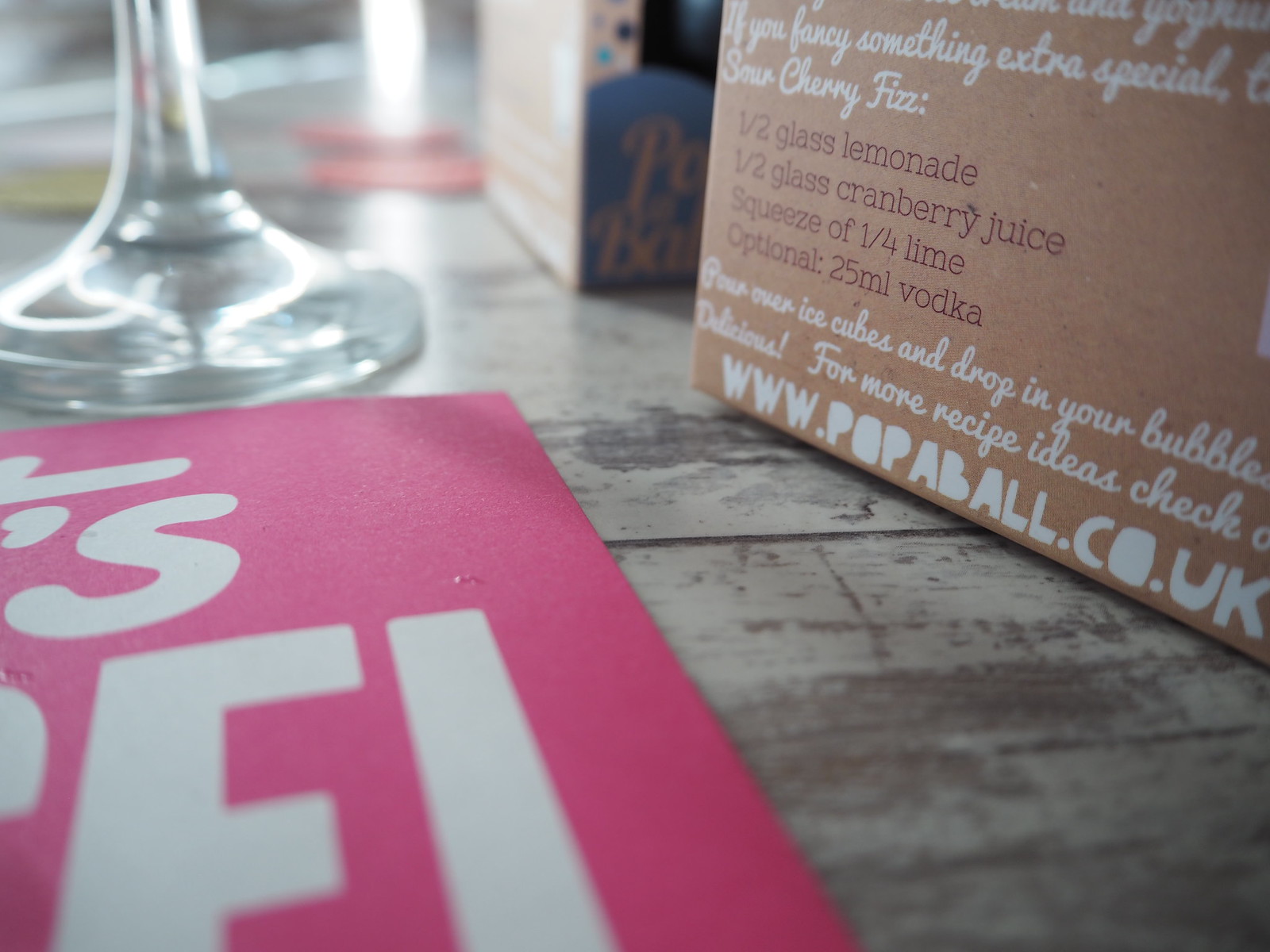In this close-up image, we're presented with a rustic, weathered wooden table, likely once brown but now largely stripped of its white paint. The table serves as the setting for various objects, suggesting an indoor environment such as a brewery or a wine tasting venue during the day. 

To the top left of the image, a wine glass glimmers, reflecting the ambient light. Directly below it, a partially cropped pink sign with white lettering adds a splash of color to the scene. On the right side, a brown cardboard box prominently displays a list of ingredients for a drink recipe: "Sour Cherry Fizz, Half Glass Lemonade, Half Glass Cranberry Juice, Squeeze of a Quarter Lime, optional 25 milliliters vodka," and a website, "popaball.co.uk," for further ideas.

The assortment of colors—pink, white, gray, brown, light brown, purple, light blue, dark blue, and orange—adds to the vibrant yet rustic ambiance of the photograph, capturing a moment of casual indulgence in what appears to be a relaxed, social setting.